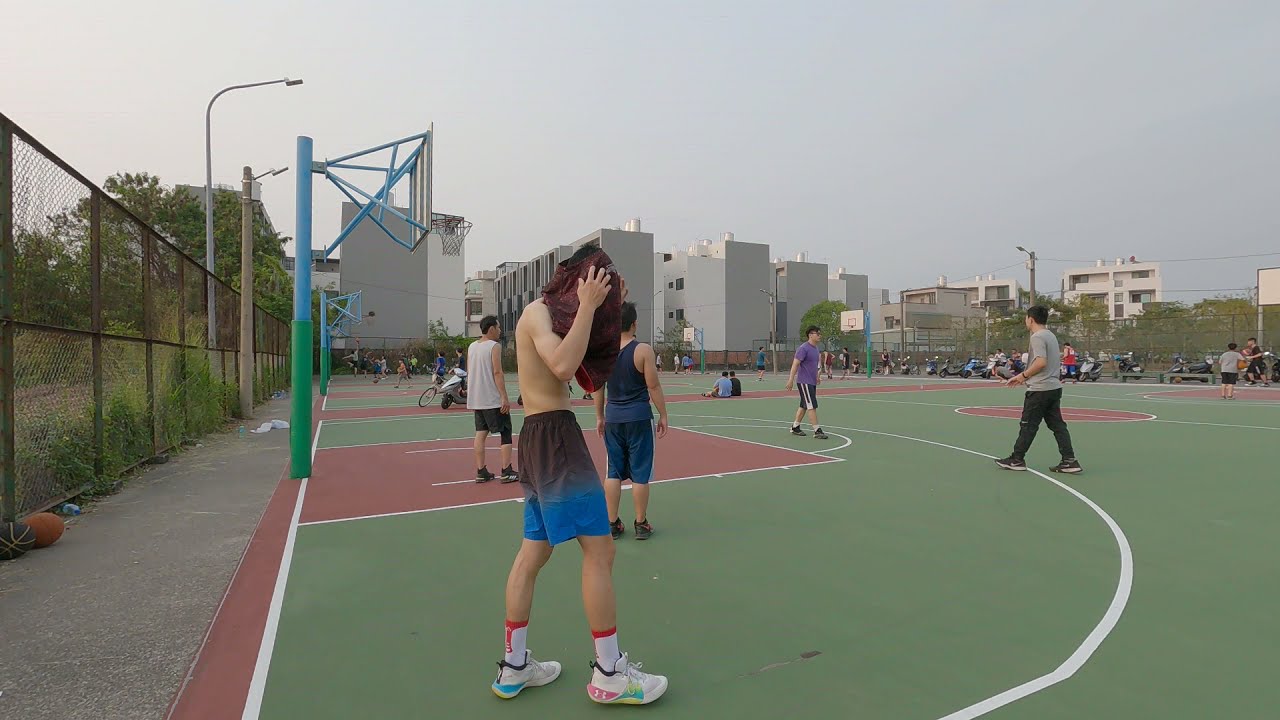This horizontally-aligned rectangular image captures a bustling scene at an expansive outdoor public recreational area dominated by multiple basketball courts. The sky overhead is mostly cloudy, presenting a blend of gray and light gray tones that cast a diffused light over the entire setting. In the background, a series of rectangular gray and white buildings, likely office buildings or apartments, frame the scene.

The central focus of the image is a large, fenced-in basketball court. Along the left side of the court, an older metal wire fence is visible. Lying on the ground near the fence, there are a basketball and a football. At the heart of the court, a young man stands shirtless, either putting on or taking off a burgundy-colored t-shirt. He is dressed in dark gray and blue shorts, white and red socks, and white tennis shoes with colorful yellow and teal accents.

Adjacent to him, a green and blue basketball hoop stands poised for play. Surrounding the shirtless young man are several other players, scattered across the court, some appearing to prepare for a game. One player nearby is wearing a blue tank top and blue shorts, while another sports black pants and a gray shirt. The court itself is detailed with the full outline and markings typical of a basketball court, featuring green flooring with red areas in the painted zones and the center court area. Farther into the background on the right, more people can be seen engaging in various games, indicating the expansive and lively nature of this recreational park.